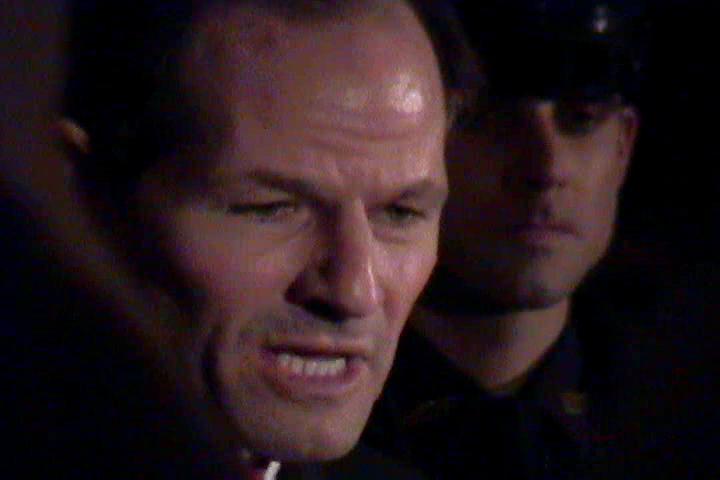The low-resolution, grainy photo appears to be a still from a movie or TV show, featuring a close-up of a white male in his late 40s to early 50s on the left side of the image. His face is partially in shadow, but a glistening shine on the top right of his face suggests some light source. He has short hair, possibly balding on the sides, with a bit of stubble around his mustache area but no full beard. He looks slightly angry or intense, with his mouth open and the bottom row of his teeth visible, as if he is speaking. He is looking down to the bottom right. To the right of him, in the background, is another white male who appears younger. This second man is dressed in what seems to be a black police uniform and hat, though the poor quality and darkness of the image make it hard to discern details. He has his eyes downcast and his mouth closed, adding to the impression that this is a dramatic scene from a visual story.